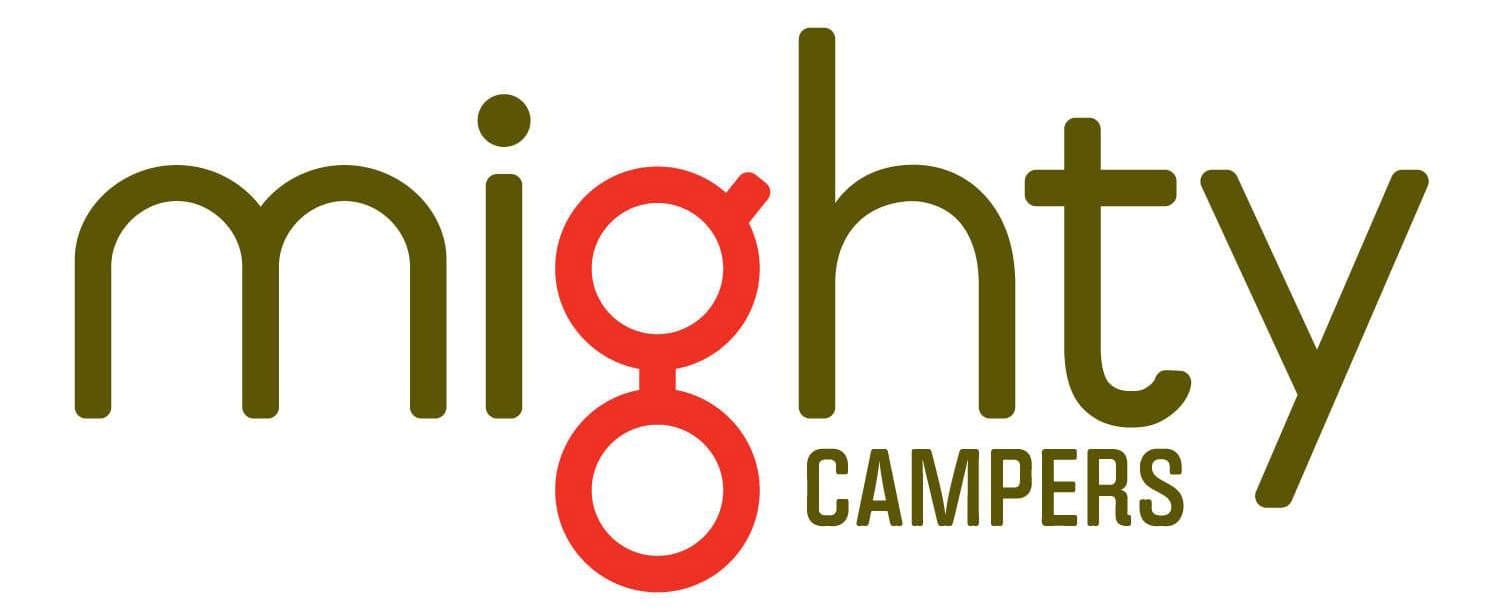The image features a digitally created logo on a solid white background. The main text reads "MIGHTY" in large letters spanning from left to right. Most letters—M, I, H, T, and Y—are colored in a dark algae green. The G is distinct, colored in red, designed as two partially overlapping circles with a small line connecting them at the top right. Below the letters H and T, in smaller capital letters, is the word "CAMPERS," also in the same dark algae green. The overall composition emphasizes the word "MIGHTY," with "CAMPERS" positioned subtly beneath it, suggesting a hierarchy in the text.